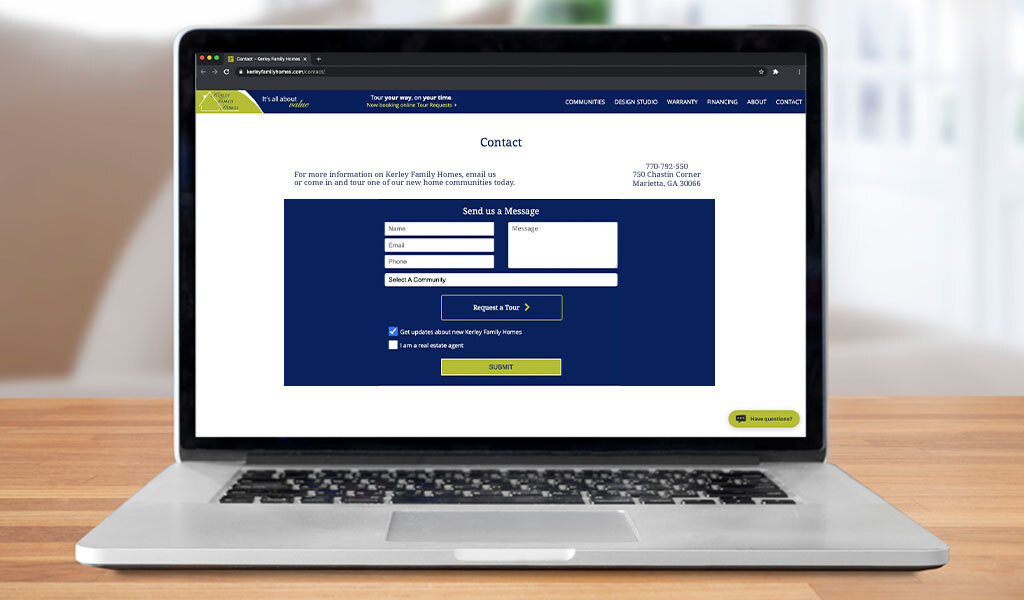This color photograph captures a close-up view of a laptop computer placed on a light brown hardwood table. The laptop itself features a silver-gray bottom surface and black keys. The screen displays a webpage with a white background. At the top of the screen, there's a navigational menu with a blue background. On the far left of this menu, there's a small section in an olive green-gold hue, although the print is too small to read clearly. The menu items are legible though, showing options like "Communities," "Design Studio," "Warranty," an undiscernible word, "About," and "Contact."

In the center of the screen, against a white background, there's a large blue rectangle, similar in color to the top menu. At the top of this white area, the word "Contact" is prominently displayed. To the right, there's a phone number and an address. Inside the large blue rectangle, several white input boxes are visible, designated for entering a name, email, phone number, and a message, indicating a contact form for user inquiries.